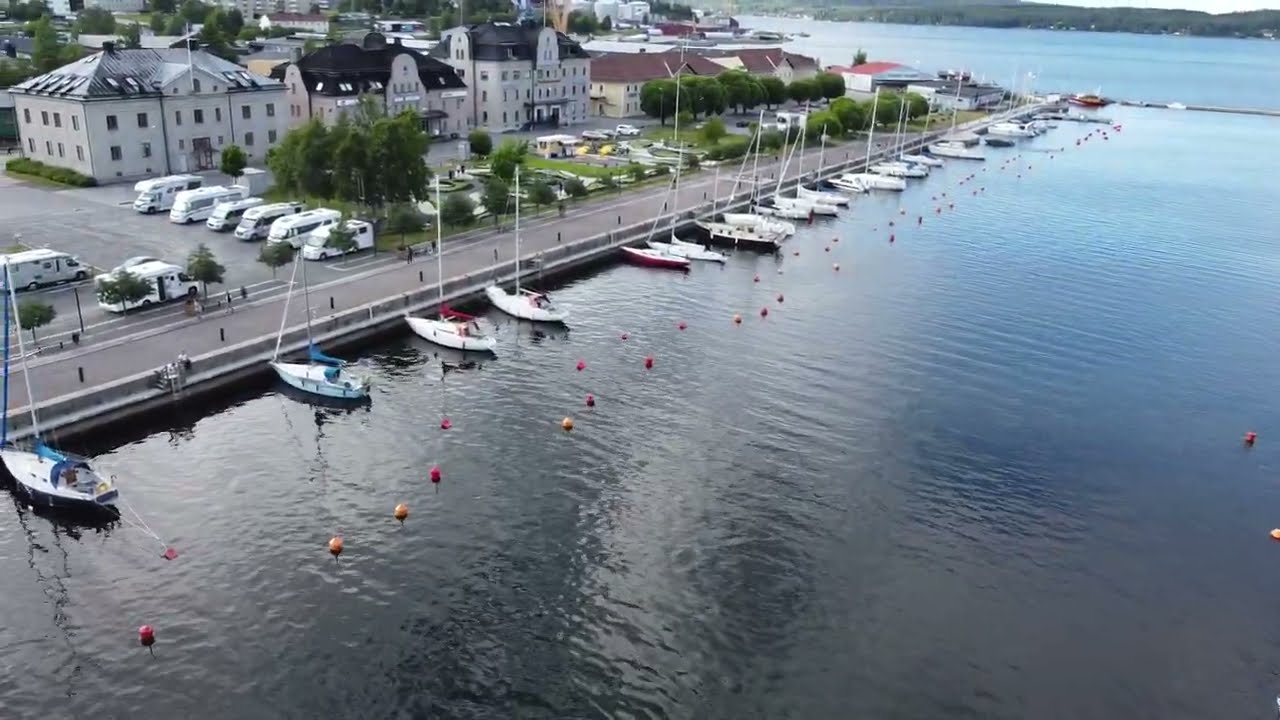The aerial image, captured from the viewpoint of a drone, showcases a striking waterfront scene. Running diagonally from the bottom left to the top right, a road lines the water's edge, creating a vibrant juxtaposition between land and lake. This road serves as a dock for an array of boats, predominantly white with varied top colors including blue, red, and black. Situated along the right side of the image, the shimmering water curves around to the background, accentuating the serene setting.

Adjacent to the dock, on the left side of the image, sits a bustling area with parked cars, vans, and several parking lots. The buildings, which appear to be primarily two-story structures with black roofs, are clustered towards the top left. In the same vicinity, a collection of shuttles and perhaps some hotel amenities suggest a well-frequented area, possibly catering to visitors and tourists.

The scene is adorned with various hues - black, red, blue, white, brown, tan, silver, and gray - highlighting the diverse elements within the frame. The setting is clearly outdoors, captured under the bright light of midday, framing a vivid and detailed tableau of a lively marina and its adjacent urban landscape.